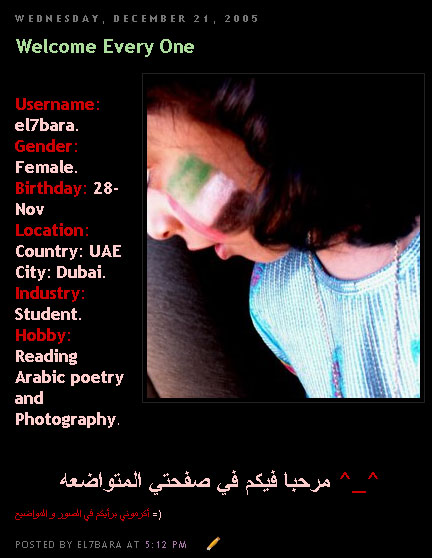The image features a detailed portrait of a young woman captured in a photograph with a black background, giving the impression of a poster design or social media profile. Her face is shown in profile with a painted emblem on her left cheek, which looks like a flag composed of green, white, and black horizontal stripes with a vertical red stripe on the left. She is adorned with a light blue silk blouse and a necklace. Above her portrait, green text reads "Welcome Everyone," accompanied by the date "Wednesday, December 21st, 2005" in white. Along the left side of the image, there is a list of personal details in a key-value format, indicating the username "EL7Bara," gender "female," birthday "28th of November," location "UAE, Dubai," industry "student," and hobbies "reading, Arabic poetry, and photography." The bottom of the image includes a single line of Arabic text in white, and there is a small pencil icon next to the time "5:12 pm" marking the post by "EL7Bara" on this date.